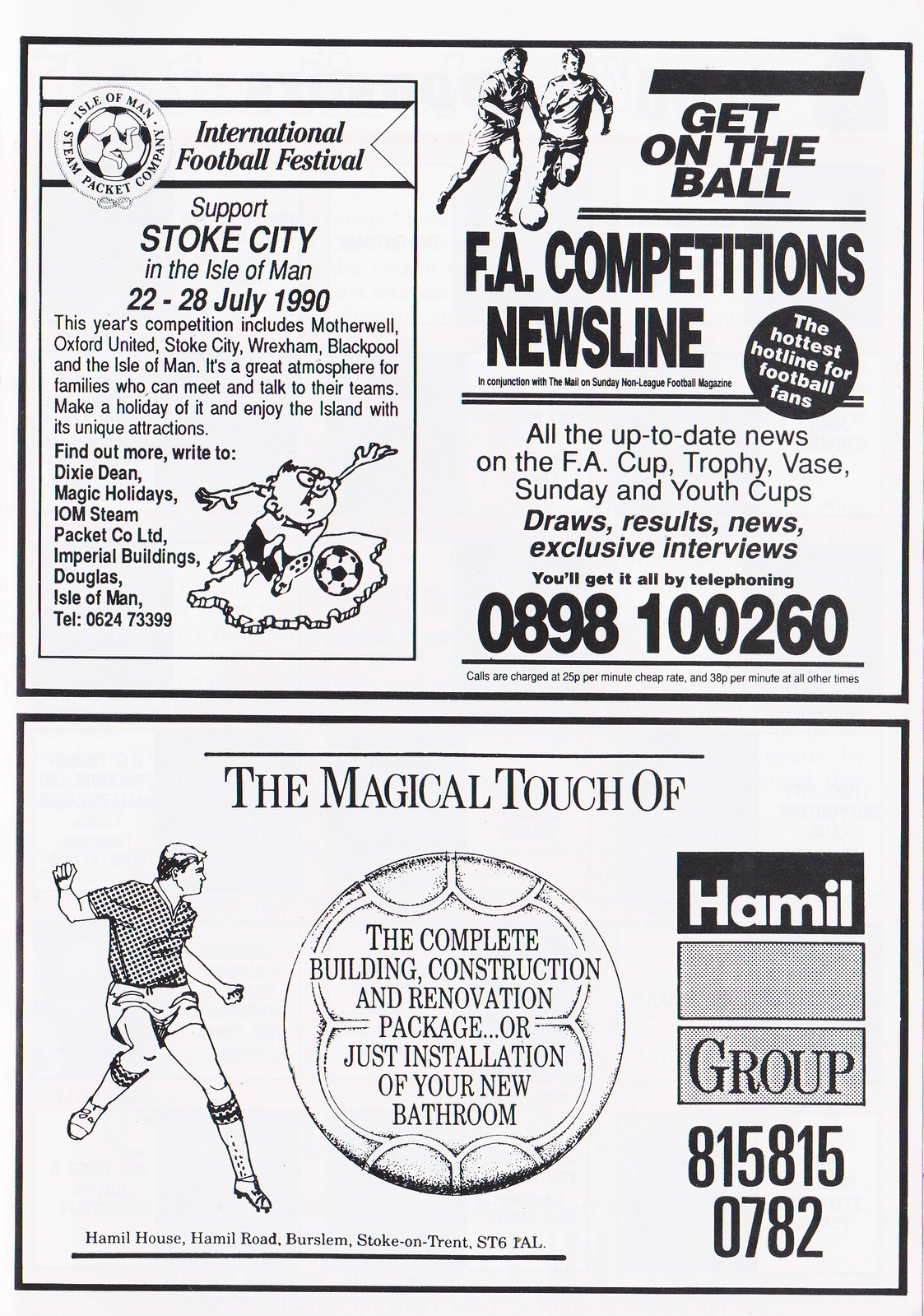This detailed black and white image resembles a magazine page featuring multiple sections. The top center showcases two soccer players vying for a ball, captioned "Get on the Ball." To the right, bold text states "FA Competitions Newsline," followed by a smaller description listing updates on the FA Cup Trophy, Vase, Sunday, Youth Cups, drawing results, news, and exclusive interviews, with a contact number, 0898-100-260. 

To the left, the "International Football Festival" announcement invites support for Stoke City in the Isle of Man from July 22-28, 1990. A cartoon image depicts a soccer player on an island running towards a ball. Below this, the text "The Magical Touch Of" leads to a 2D soccer ball with a message, "The Complete Building Construction and Renovation Package, or Just Installation of Your New Bathroom."

An additional soccer player image, one foot raised and arms in motion, is also present, looking towards the image center. The Hamill Group logo, featuring three squares—one black with "Hamill" text, the others checkerboard—appears at the bottom right with the number 815-815-0782. Below in small print, "Hamill House, Hamill Road, Burlem Stoke On Trent, ST6, FAL" reads in black text against a white background.